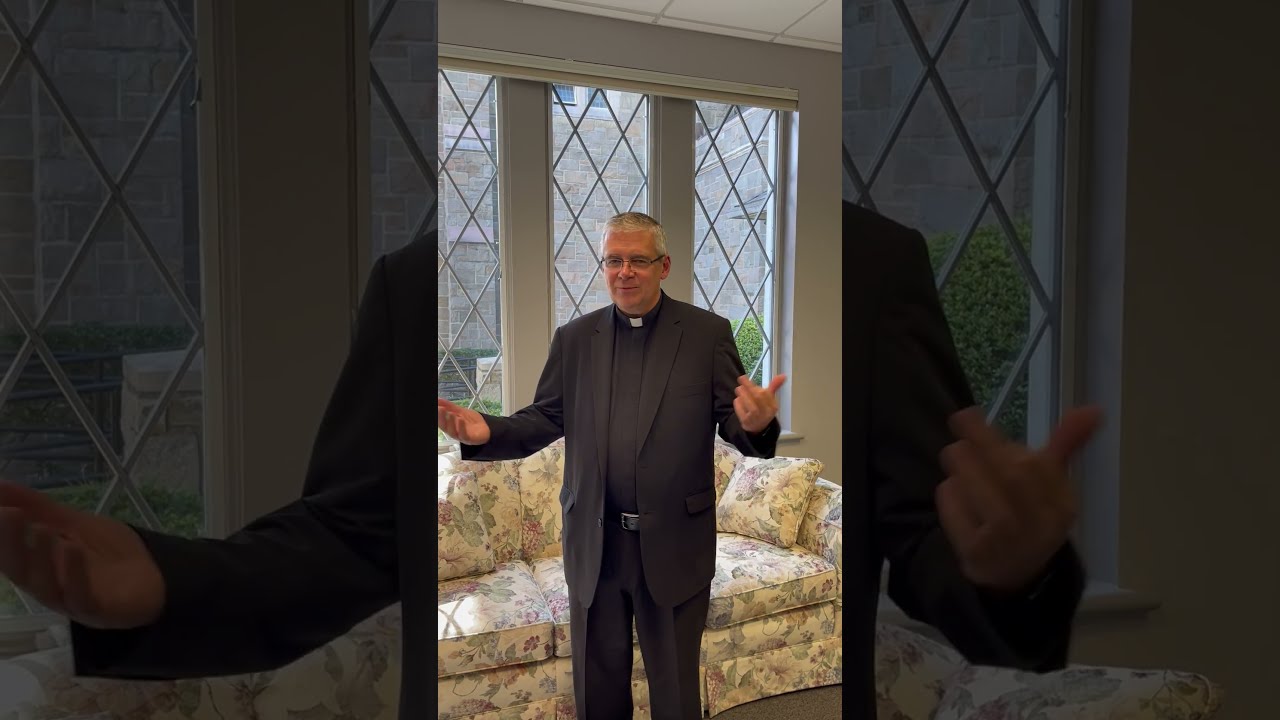This image is divided into three segments, with the outer right and left segments darkened by a filter. The central segment features an older Catholic priest with predominantly gray hair, wearing glasses. His attire includes a black jacket, a black button-up shirt, a silver-buckled belt, and black pleated pants, along with the distinctive white Roman collar. The priest's arms are extended out to his sides with palms up, and he appears to have a slight smile while looking down. Behind him is a cream-colored floral couch and three windows with diamond-shaped panes. Through these clear, leaded glass windows, a brick wall with additional windows is visible. The location has light gray walls, a ceiling of white tiles, and a light gray carpet. The outer segments of the image feature blown-up, darker versions of the priest's arms.